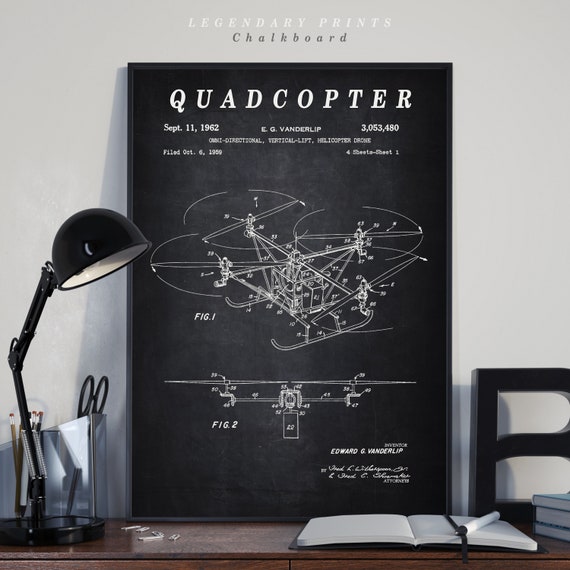The photograph, perfectly square in shape, captures a desk scene centered around a large poster meticulously detailed and framed in a commercial setting, likely to entice buyers. Dominating the scene, the poster features a prominent black background with the intricate diagram of a quadcopter, identified by its four distinct rotors. White text on the poster reads: "Quadcopter, September 11th, 1962, E.G. Vanderlift, 3,053,480 Omnidirectional Vertical Lift Helicopter Drone Filed October 6th, 1956." Above this poster, the wall bears white text proclaiming "Legendary Prince" followed by the black text "Chalkboard." Anchoring the scene is a dark wooden desk, upon which the poster is displayed. To the left, a movable black table lamp stands hinged and adjustable, flanked by a pencil and scissors container. On the right side of the desk, an open notebook with a pen rests strategically, beside a stack of books partially out of view. The desk is positioned against a pale blue wall, enhancing the composition with a calm backdrop.